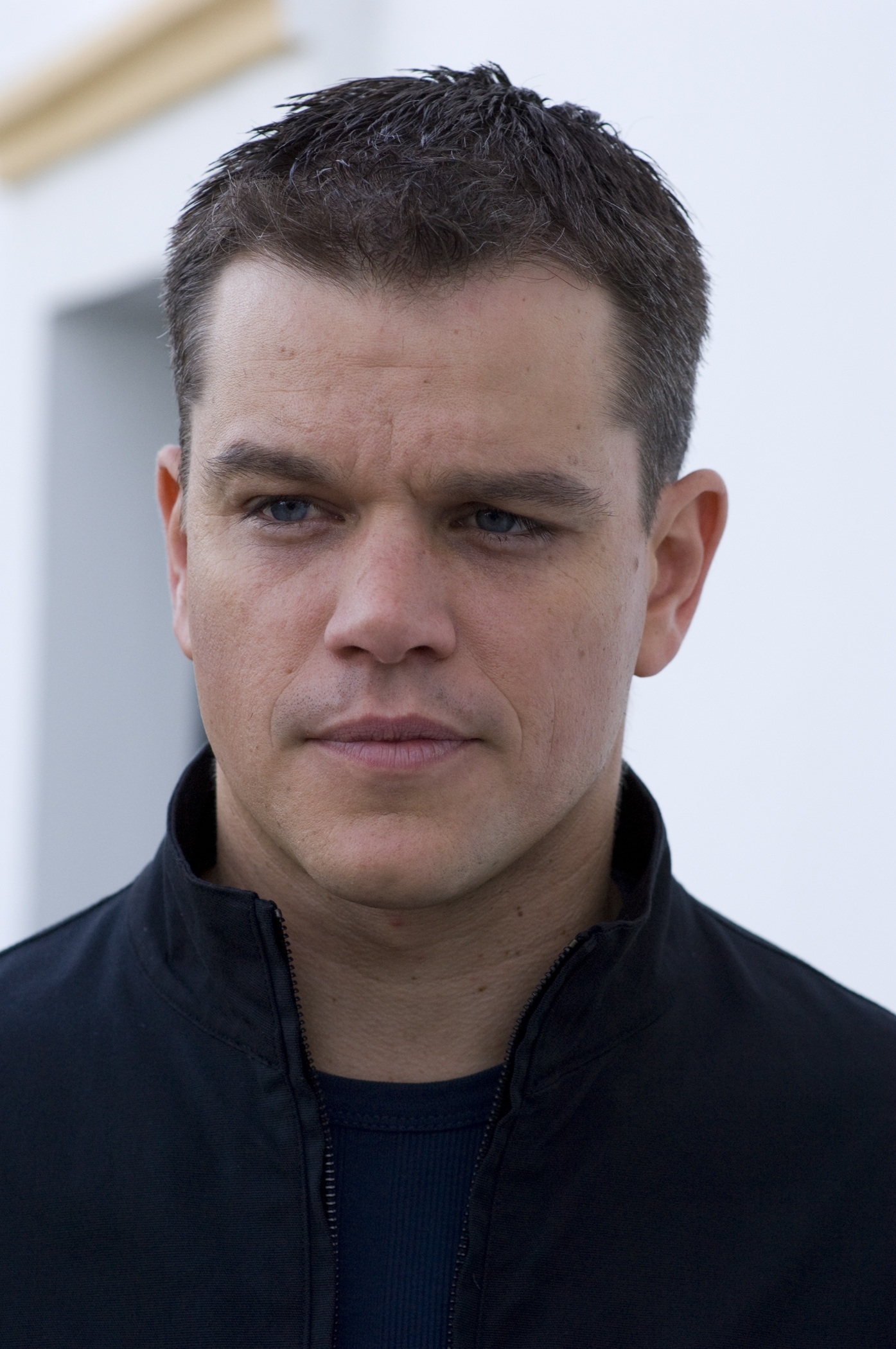This is a vertical, rectangular photo of actor Matt Damon. He has very short dark brown hair and blue eyes, and he appears clean-shaven with only a slight mustache shadow. Matt is looking off to the side with his eyebrows scrunched, displaying a straight, slightly serious expression. He is wearing a navy blue t-shirt under a black zip-up jacket with a collar. The image captures him from the shoulders up against a blurred background with a white wall and a faint outline of a building. Subtle wrinkles are noticeable on his face, especially around his scrunched eyebrows.